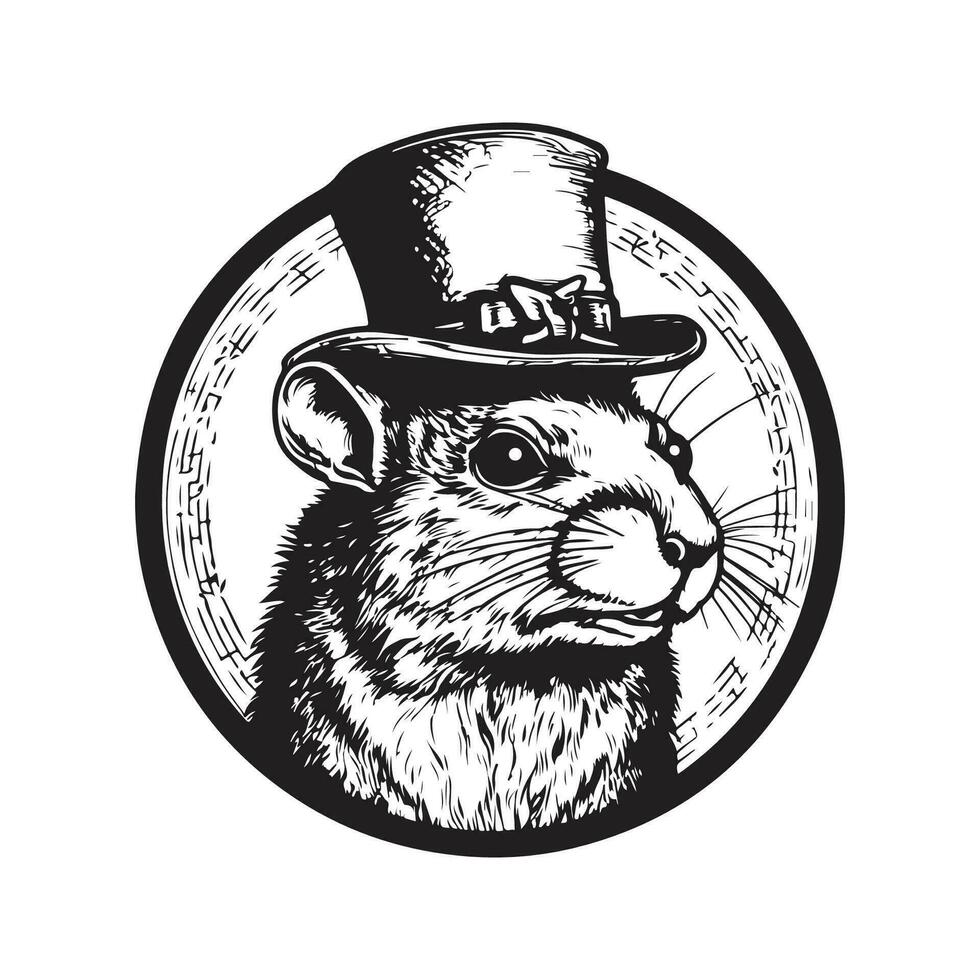The image presents a centrally placed, detailed illustration against a white background. The main subject is a circular, heavily bordered button or disc adorned with intricate etchings. Inside the circle is a finely detailed animal, primarily identified as a gopher but with features that might suggest a dormouse or rat. This creature is depicted with dark, expressive eyes, visible black-tipped whiskers, and long upper eyelashes. Its mouth, slightly parted beneath a cat-like nose, reveals no teeth. The gopher wears a tall top hat adorned with a distinct ribbon or belt around its base, with part of the hat slightly extending beyond the confines of the circle. The hat's design suggests a possible association with St. Patrick's Day or a political campaign, given its notable features and style. The background within the circle is filled with a pattern of circular lines, adding depth and texture to the overall illustration.